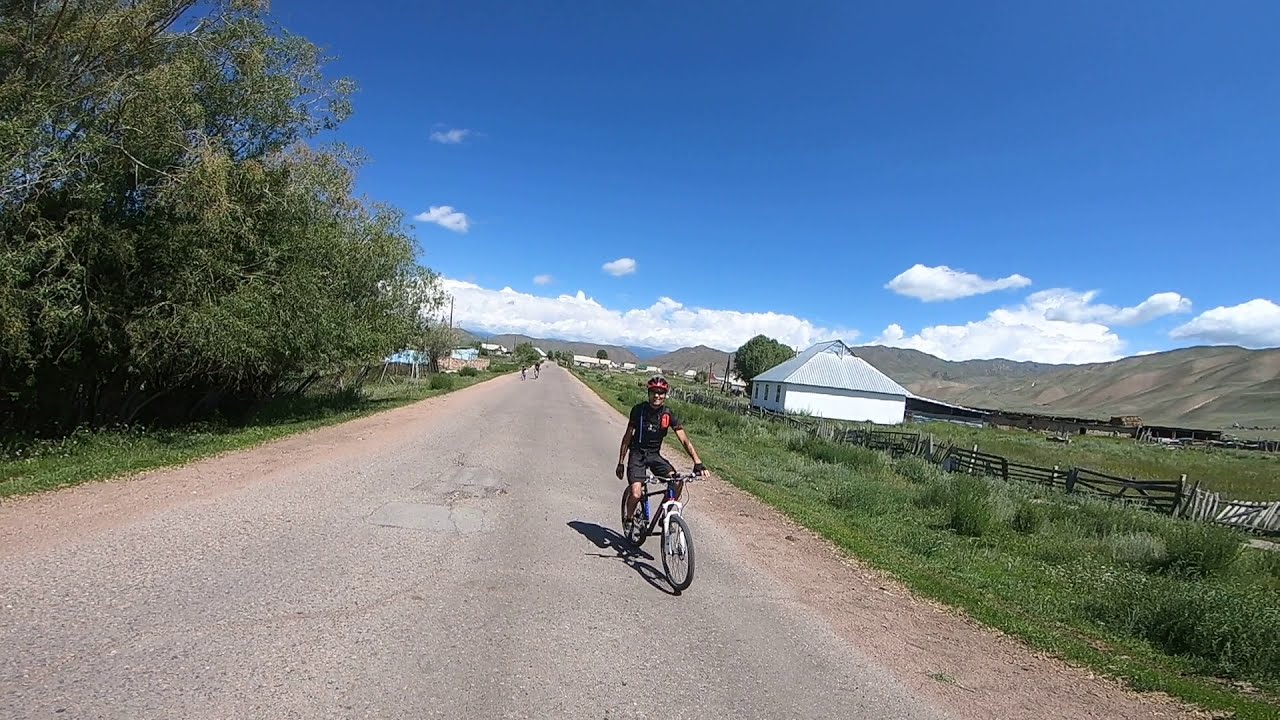In this wide rectangular photograph, a man is cycling towards the camera in the center of the image, dressed in a black and red uniform with a matching helmet, riding a white bicycle. The cement-gray road he is on converges towards the horizon line in the middle of the photograph, creating a sense of depth. The left side of the road is lined with tall, messy green trees and grass, while the right side features uncut grass, a wooden fence, and a white barn in the distance, indicating a rural, farm-like setting. Additional cyclists can be seen in the distance on the road behind him. The horizon is marked by a range of mountains on the right side of the image. The sky above is a bright blue, adorned with thick white clouds at the bottom where it meets the horizon, enhancing the scenic and peaceful atmosphere of this rural landscape.